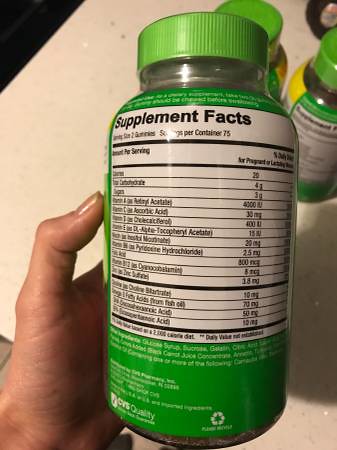A detailed photo showcases a person's left hand holding a bottle of supplements. The hand and thumb firmly grip the plastic bottle, which features a green cap and a white label. The label, illuminated by bright light, details the supplement's contents, indicating it provides nutrition for two gummies and offers 75 servings per container. The label also lists various vitamins, minerals, and their respective dosages. The background reveals an off-white table, adorned with several other bottles, each equipped with green caps and green labels, further emphasizing the supplement theme. The composition highlights the intricacies of the label while situating it within a context of similar products, suggesting a focus on health and wellness.